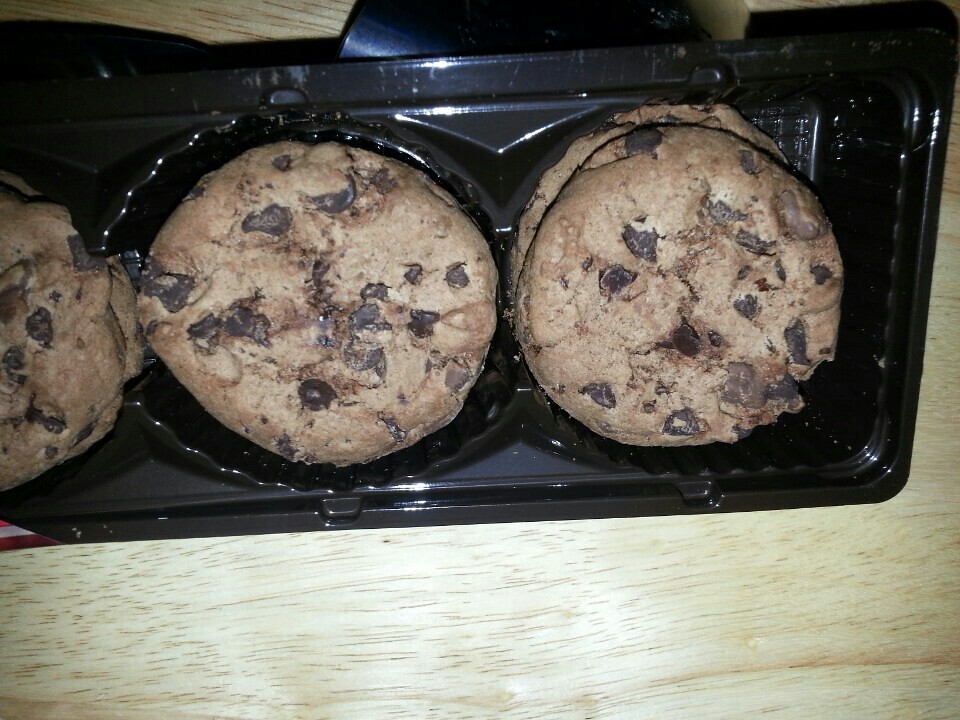The image shows a freshly opened plastic container with six chocolate chip cookies, neatly arranged in three small trays. The long, square container, made of very dark black plastic, is designed specifically to hold these cookies, with each tray accommodating two cookies. The cookies are baked to a golden brown color, with numerous chocolate chips visibly melted into them, making them look delicious. This black plastic container rests on a wooden table, adding a rustic touch to the presentation.